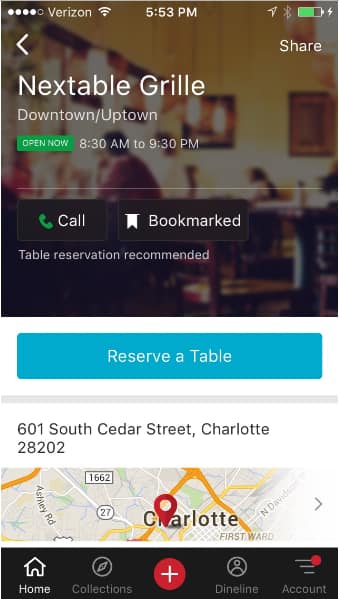Screenshot of a smartphone displaying the order page for "Nextable Grill." The status bar at the top shows a Verizon signal with four to five dots, a full Wi-Fi signal, the time as 5:53 PM, location and Bluetooth icons, and an approximately 70% battery level. Navigation icons include a back arrow on the left and a share option on the right.

The order page text is overlayed on a blurred background of a cafe or coffee shop with yellow walls and pendant lights, creating an intentional blur to highlight the text. The page has been darkened slightly to enhance text readability. 

The header reads "Nextable Grill," followed by the location indicator "downtown/uptown." A green button indicates the restaurant is "Open now" with operating hours from 8:30 AM to 9:30 PM. Below this, a thin white line separates the header from two action buttons: a green "Call" button with a phone receiver icon and a gray "Bookmark" button indicating it has been bookmarked. An advisory note suggests, "Table reservation recommended."

A large light blue button at the bottom of the screen, almost spanning the width of the phone, prompts users to "Reserve a table." Directly beneath this button is the address "601 South Cedar Street, Charlotte, 28202," displayed above a sliver of an interactive Google Maps section.

At the very bottom of the screen, a navigation menu includes tabs labeled "Home," "Collections," "Plus," "Dine," and "Account."